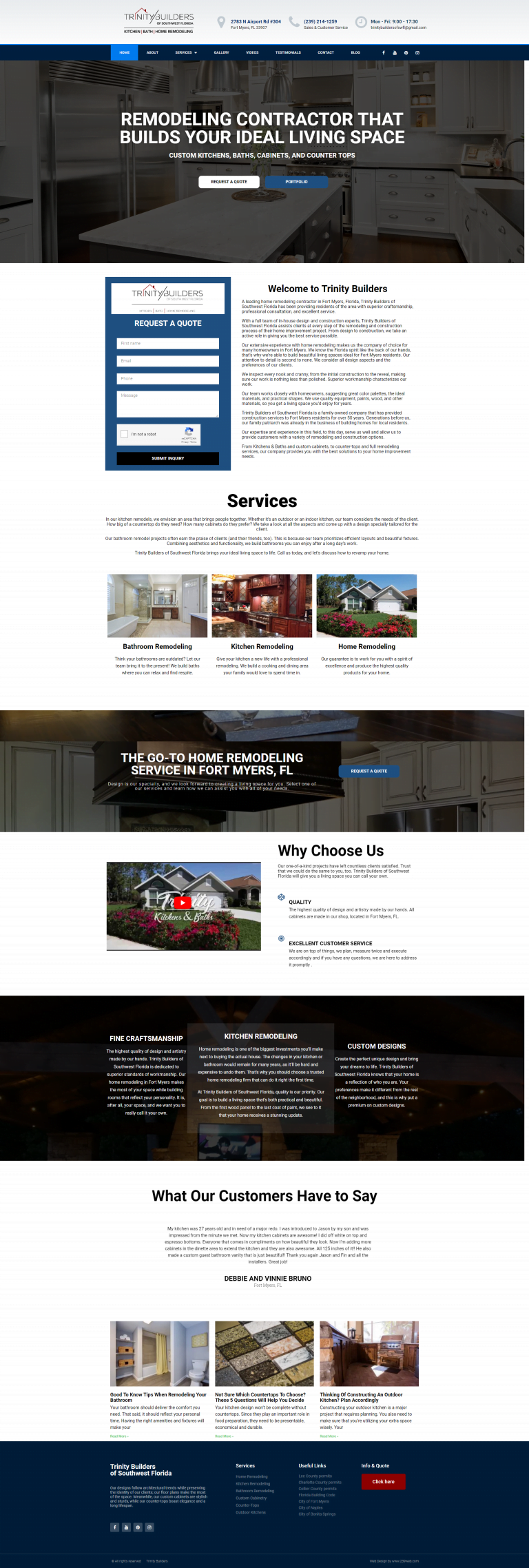This is a highly zoomed-out screenshot of a website, making it challenging to see details clearly. At the top of the page, large, white text is prominently visible, reading "Remodeling Contractor That Builds Your Ideal Living Space." Directly below this text, the site features two buttons: a white one on the left and a dark blue one on the right.

Further down, there is a large black section labeled "Our Services," under which there are three separate images, presumably representing different services offered by the company, although the details are hard to discern due to the zoomed-out view.

Below this section, there is a dark background banner with white text, which appears to state, "The go-to home remodel service in Fort Myers, Florida." Following this banner is a section titled "Why Choose Us," likely highlighting the company's credentials and past accomplishments.

The final section visible in the screenshot is labeled "What Our Customers Have to Say," which seems to be a review section featuring testimonials and personal experiences from previous clients.